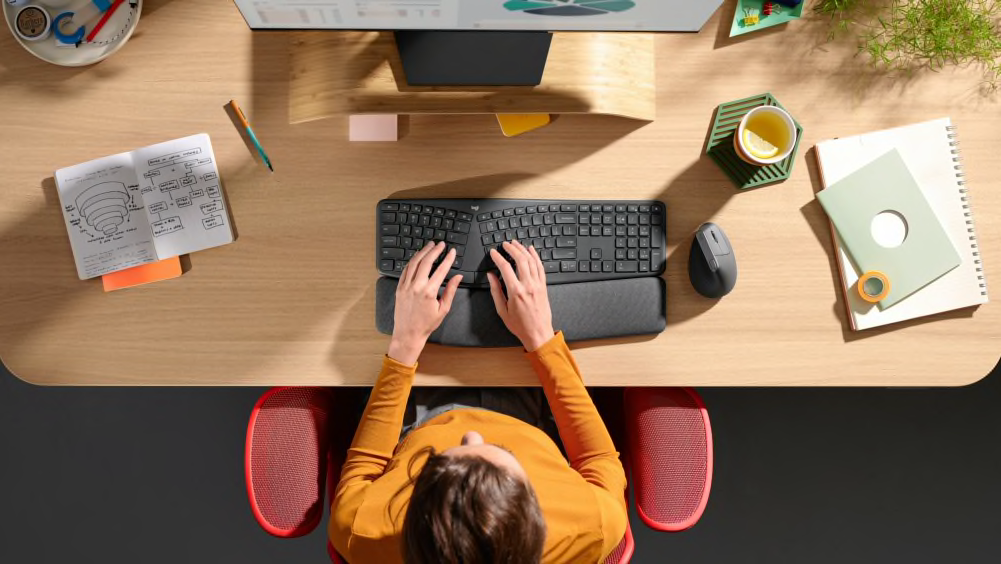This detailed aerial view photograph captures a brown-haired Caucasian man, seated in a red mesh office chair at a light faux wood desk. He is dressed in a russet long-sleeved shirt and is actively using an ergonomic black keyboard with a wrist cushion, positioned in front of a slightly cropped computer screen displaying what appears to be pie charts. On the immediate right of his keyboard is a dark gray wireless mouse, and a hexagonal silicone mat potentially holding a cup of coffee or juice. To his right lies a spiral notebook, and to his left, a manual with notes and drawings, accompanied by an orange marker and a pen. The desk surface also features a bamboo stand lifting the computer monitor, under which are some sticky notes. An asparagus fern in the upper right corner adds a touch of greenery, while a dish containing unclear items sits in the upper left corner.